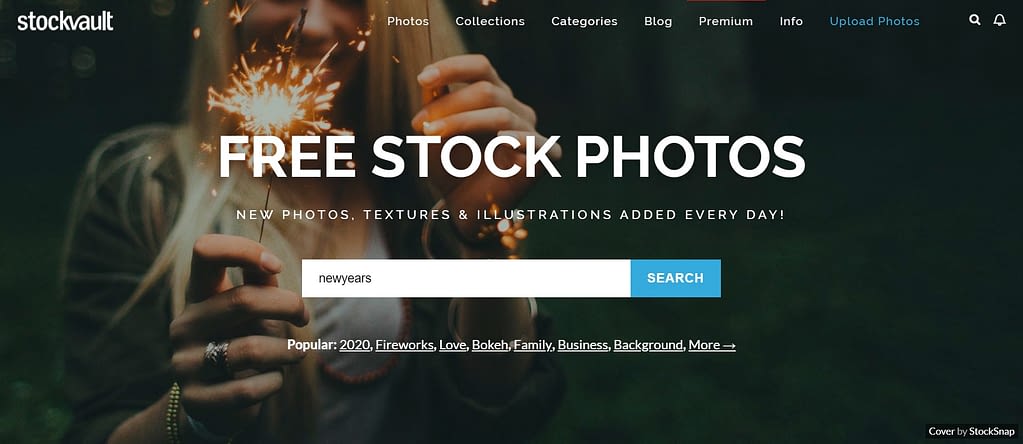This screenshot portrays a desktop user interface with a celebratory theme. The background showcases a partially cropped image of a Caucasian woman with long, straight blonde hair, visible from the nose down. She is holding sparklers in both hands, with the sparklers in her left hand extending beyond the bottom of the frame. Adorning her left hand, she wears a silver ring on her ring finger and silver bracelets.

Her attire includes a khaki-colored upper garment with a white undershirt visible underneath. Overlain on the image, in large white text across the central part of the page, are the words "Free Stock Photos." Directly beneath, in smaller text, it reads, "New photos, textures, and illustrations added every day."

A prominent white search box is centered below this text, with the placeholder "New Year's" inside. To the right of the search box, there is a blue search button labeled "Search." Underneath the search functionality, there's a section marked "Popular," listing links such as "2020," "Fireworks," "Love," "Bakerly," "Family," "Business," "Background," and "More," followed by a right-facing arrow.

The top left of the screen features the logo and title "StockVault," indicating the website's name. The header includes navigation links for "Photos," "Collections," "Categories," "Blog," "Premium," "Info," and "Upload Photos," providing various resource and functional options for users.